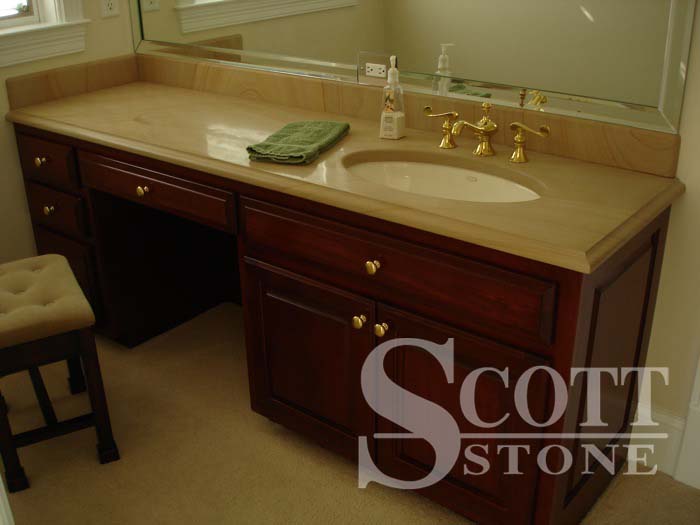This image showcases a meticulously arranged vanity area that has been cleverly crafted from a cabinet and sink setup. A large mirror spans the wall above the counter, reflecting an airy and functional space. Centrally positioned on the countertop, a pump soap dispenser sits adjacent to an electrical outlet. In front of the outlet lies an olive green hand towel, adding a touch of color to the scene.

The countertop features a dark cream, tan-ish hue that harmonizes beautifully with the brass faucet and dark cherry wood cabinetry beneath. Adjacent to the sink area is an integrated desk, perfect for getting ready in the morning. The desk incorporates a small pull-out drawer and ample space for a chair. On one end, there are three or four drawers, providing additional storage.

To the right of where the chair would fit, another outlet is mounted on the wall, alongside a partially visible window that lacks curtains. The room appears carpeted, adding to its comfort and warmth. Finally, the chair itself is a tan cushioned seat with a cherry wood base, matching the cabinetry and contributing to the cohesive design of the space.